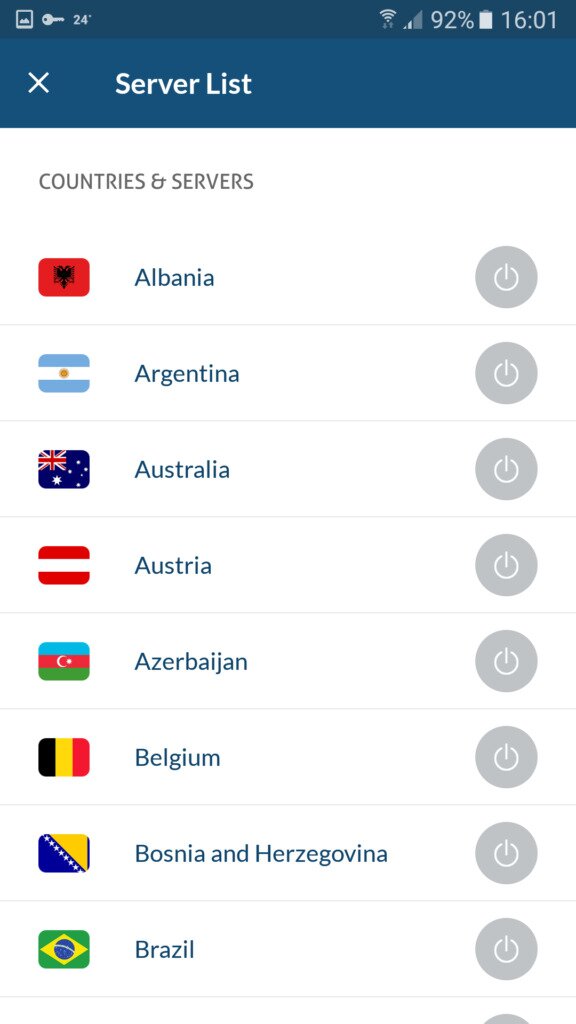This image is a screenshot of a phone screen displaying a server list for a VPN or similar service. At the top of the screen, there's a blue banner with a white text header reading "Server List." In the top left corner, an image icon, a key icon, and a temperature reading of 24 degrees are visible. On the top right, there are icons for cellular service, Wi-Fi, and a battery level at 92%, with the time shown as 16:01.

Below the "Server List" banner, there's another header in gray text that says "Countries and Servers." This is followed by a list of countries, each accompanied by its national flag on the left and a power button icon on the right. The visible countries and their corresponding flags are:

1. Albania - Red flag with a power button to the right.
2. Argentina - Teal and white flag with a power button to the right.
3. Australia - Australian flag with a power button to the right.
4. Austria - Red and white flag with a power button to the right.
5. Azerbaijan - Azerbaijani flag with a power button to the right.
6. Belgium - Belgian flag with a power button to the right.
7. Bosnia and Herzegovina - Bosnian flag with a power button to the right.
8. Brazil - Brazilian flag with a power button to the right.

The list appears to be scrollable, as there's a partial view of another power button at the bottom, hinting at additional entries below the visible portion.